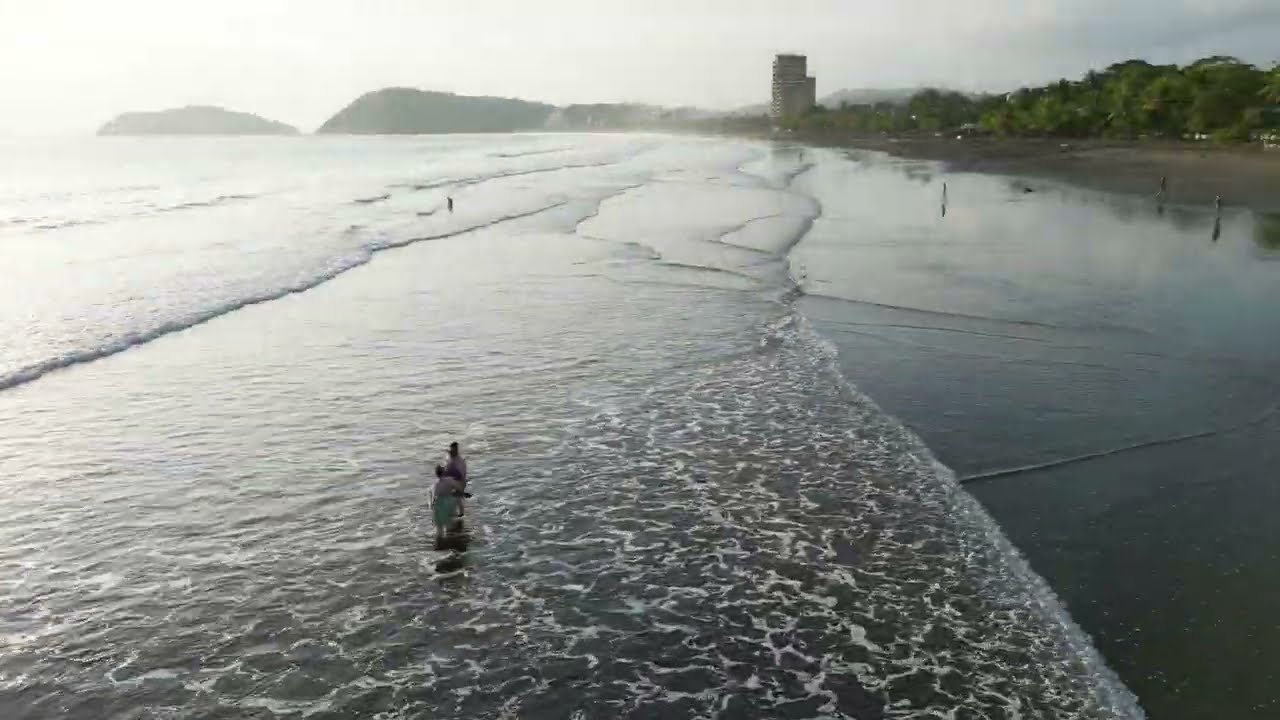The photograph captures an elevated view of a seashore where the coastline, beach, and ocean converge. On the left side, the sea dominates with gray and white colored waves creating white ripples as they hit the beach. Several people are standing in the water; notably, there is a couple near the bottom-left middle, with more individuals scattered to the upper right, including one person further out into the tide. The beach, stretching on the right, is wide and sandy, populated with many beachgoers. Water flows around some people's legs due to incoming waves. Further right, a green tree line is visible, providing a buffer space before the beach stretches toward a distant tall building structure. Beyond the building, some short hills rise in the far background. The sky above is overcast and gray, suggesting an impending storm.